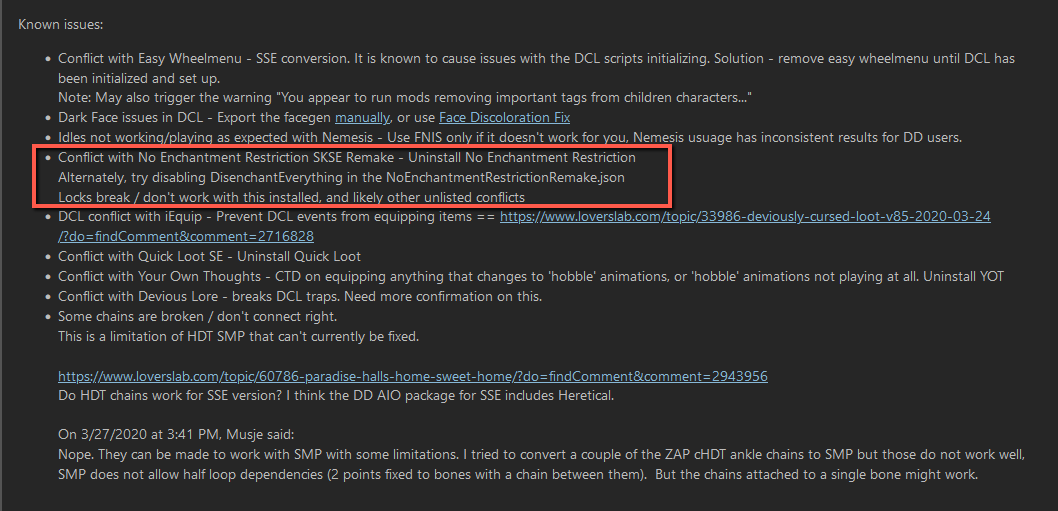**Caption:**

The image features a black background with a long horizontal rectangle shape. The text within the image is mostly in gray font and is centered, offering a detailed list of known issues and their solutions. 

**Known Issues:**

- **Conflict with Easy Menu Wheel (Menu SSE):** Known to cause issues with the DCL script initialization.

  **Solution:** Remove Easy Menu Wheel until DCL has been fully initialized and set up.

- **Warning Trigger:**

  **Message:** "You appear to run mods removing important tags from children characters..."

- **Dark Face Issues in DCL:**

  **Solution:** Export the facegen manually (word 'manually' underlined in blue) or utilize the Facegen Coordination Fix (also underlined in blue).

- **Idles Not Working/Playing as Expected with Nemesis:**

  **Solution:** Use FNIS (in all capitals) if Nemesis provides inconsistent results for DD users.

**In Red Text and Outlined in Red Rectangles:**

- **Conflict with No Enchantment Restrictions SKSE Remake:**

  **Solution:** Uninstall No Enchantment Restrictions or disable "Disenchant Everything" in the No Enchantment Restriction Remake JSON.

  **Additional Note:** Lock breaks/don't work with this installation and may cause other unlisted conflicts.

This well-structured caption highlights each issue with suggested solutions, emphasizing the text for clarity and ease of reading.